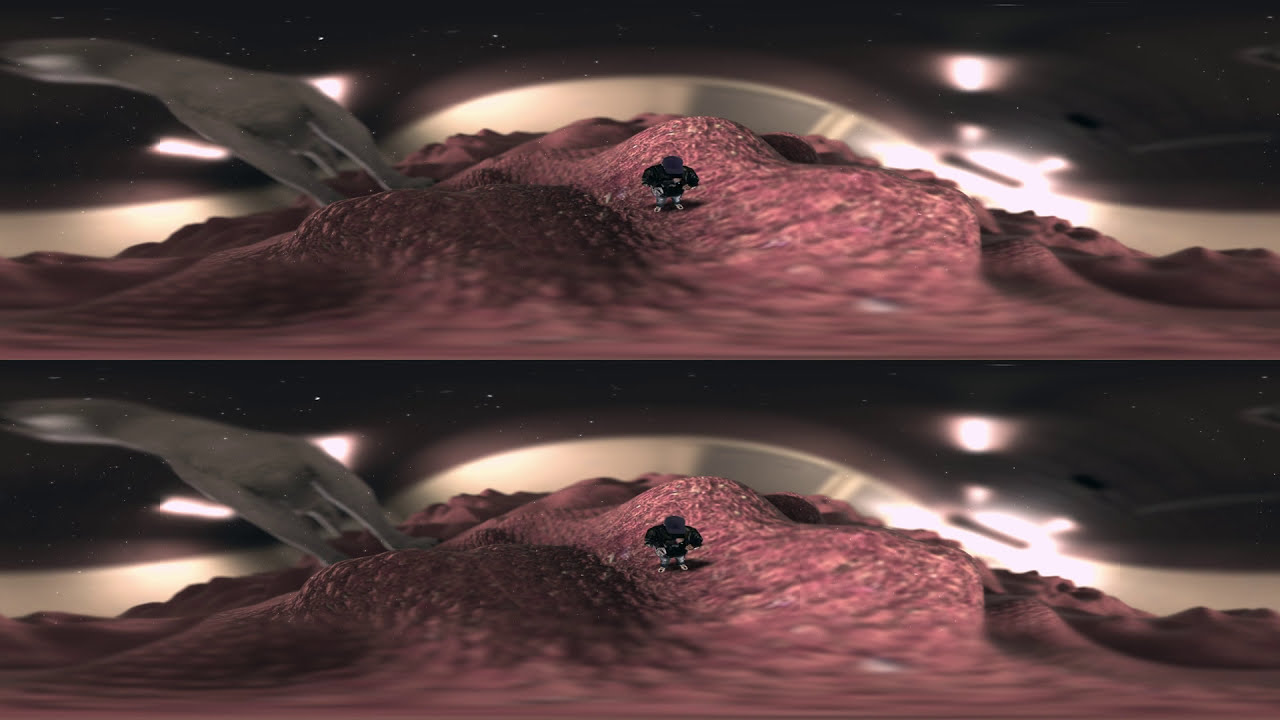The image is composed of two identical rectangular sections, one on top and one on the bottom, giving it a mirrored effect. Both sections depict a dark black sky with scattered white stars, and beneath it lies a landscape that appears otherworldly. The terrain is a textured, reddish-pink color, with numerous lumps, bumps, and varied slopes creating a sense of depth and contour. A central white stripe or mountain-like shape stretches horizontally across the image, backed by what seems to be a mound of rock.

On the left-hand side, there's an oddly shaped dark gray structure resembling three fingers, the middle one being notably shorter, which might be reminiscent of a distorted wrist. Another prominent feature in the landscape is a peculiar object that might resemble a walking cartoonish person or a small black robot, situated in the central valley between the two red hills. Additionally, there's a silver protrusion on the left side, along with other amorphous shapes that vary in color, including hints of green and dark brown. Together, these elements create a surreal landscape that could be likened to an alien planet's surface.